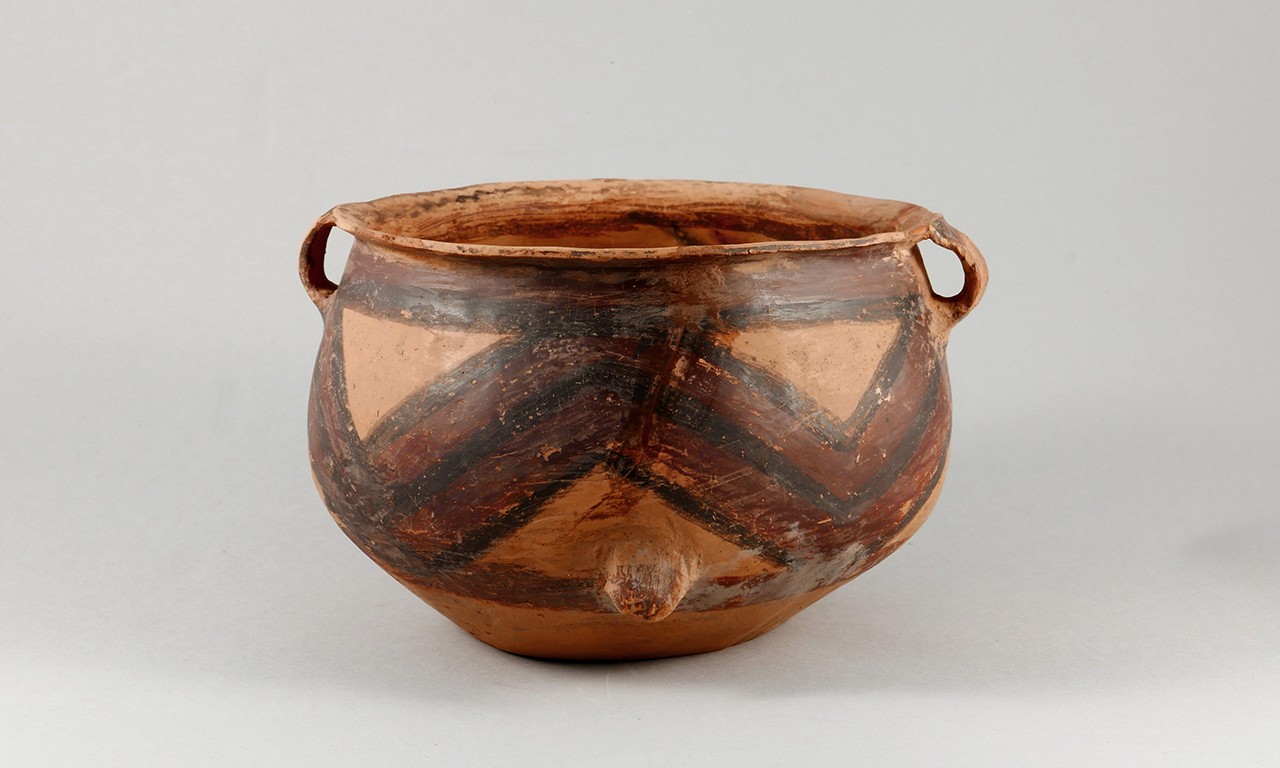The photograph is of a very old bowl that appears to be made of clay, possibly dating back to ancient Greek or Roman times. The bowl is round and measures approximately 8 to 10 inches in diameter. It features two small handles on either side, each of which can accommodate about two fingers for lifting. The bowl is predominantly brown with a painted design: there are two brown bands, one at the top and another at the bottom, connected by a W-shaped pattern in between. On the front of the bowl, there is a protruding knob, which could be a decorative element or a result of the pottery process. The detailed geometrical design and the overall appearance suggest it's a meticulously crafted piece, reminiscent of those you might encounter in a museum. The background of the photograph is gray, providing a neutral contrast that highlights the intricate details and craftsmanship of the ancient bowl.